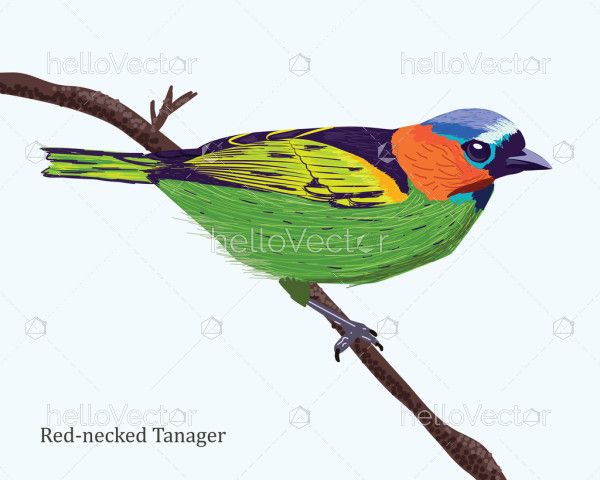This is a detailed and vibrant drawing of a red-necked tanager perched on a brown, speckled twig that extends from the upper left to the bottom right of the image. The bird is facing to the right and showcases a striking array of colors. It has a blue forehead and a blue beak, with light blue around its eyes. The top part of its neck is vivid orange, transitioning to blue and teal blue under its neck. Its back is adorned with purple and yellow hues, while the wings display yellow-green streaks. The tanager’s abdomen is green, and its tail is a mix of purple and green. A deep blue or black stripe runs down its back. Superimposed faintly over the surface of the white background are the words "HELLO VECTOR," the logo of a stock image company. In the very bottom left corner, "RED-NECKED TANAGER" is inscribed in light green letters.